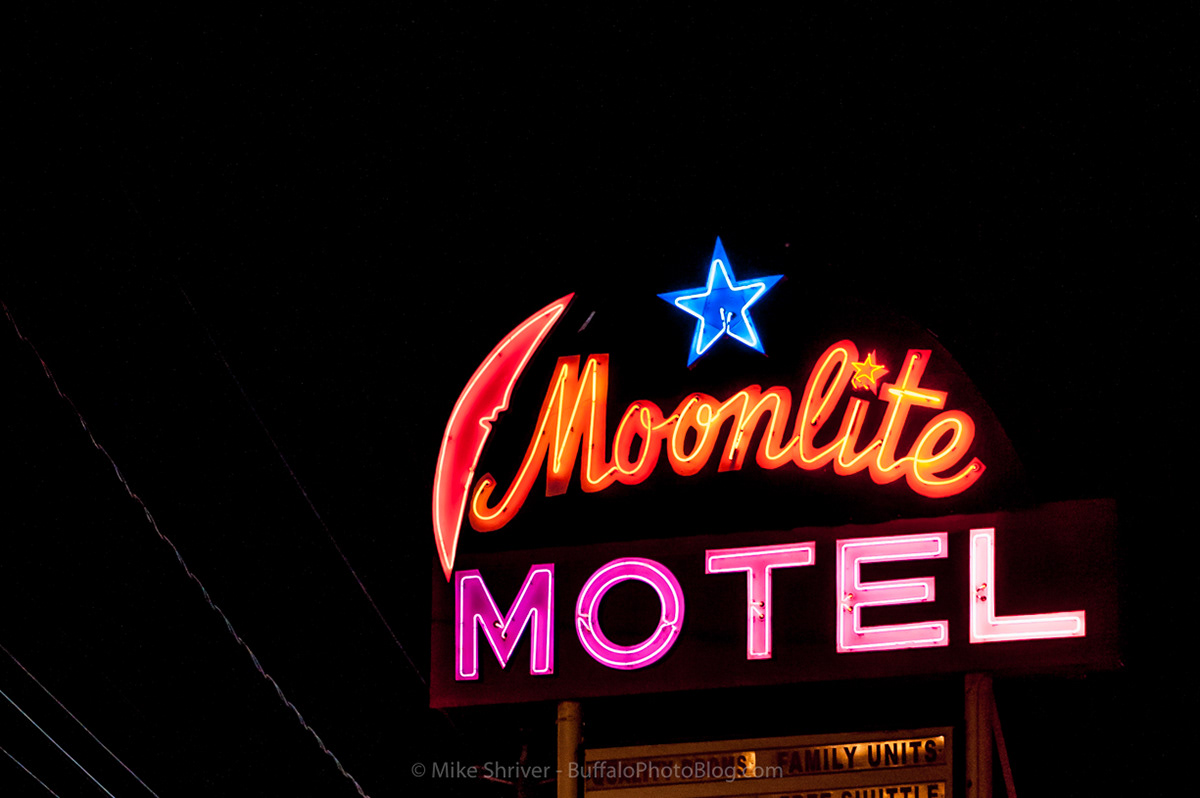This photograph captures a striking nighttime scene centered around a neon sign for a hotel against a pitch-black sky. The main feature is the vibrant 'Moonlight Motel' sign. At the very top, a neon blue star sits prominently above the rest. Below the star, the word "Moonlight" is written in cursive with a neon orange glow, flanked by a red crescent moon on the left. Beneath "Moonlight," the word "MOTEL" appears in all capital letters in bright purple neon block letters. The illuminated sign continues downwards to a backboard dimly lit with black writing, where only the words "family units" are distinctly visible on the top right of the board. Additionally, on the lower left, a few white streaks, probably reflecting telephone or power lines, are visible. At the very bottom center of the photograph, there’s a watermark that reads "Mike Shriver, buffalophotoblogs.com."